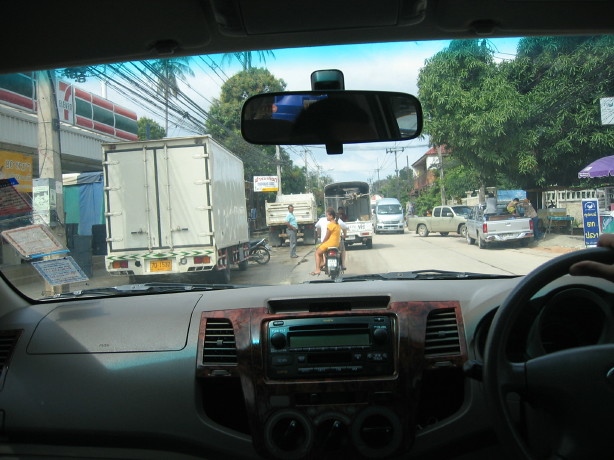In this color photograph taken from the back seat of a right-hand drive vehicle, the focus is looking through the windshield onto a bustling street scene. To the immediate front of the vehicle, a person in a white short-sleeve t-shirt rides a motorcycle with a girl dressed in an orange-yellow short-sleeve outfit and short trunks sitting sideways behind them. Directly ahead, a bus appears to be moving in their direction, indicating active traffic flow. On the right side of the street, a couple of trucks, potentially semis or box trucks, are parked, with a man in blue jeans and a blue top standing nearby. Further up the right side, a vibrant green tree and a colorful blue and purple umbrella add to the urban setting. To the left, off the road, a storefront displays the familiar orange, green, and red logo of a 7-Eleven store. Additional details include power lines stretching overhead, blue signs, and a gray van coming from a distance, contributing to the busy, city street atmosphere. The road itself appears to be packed gravel or dirt, emphasizing the scene's rustic charm encapsulated within a cityscape.